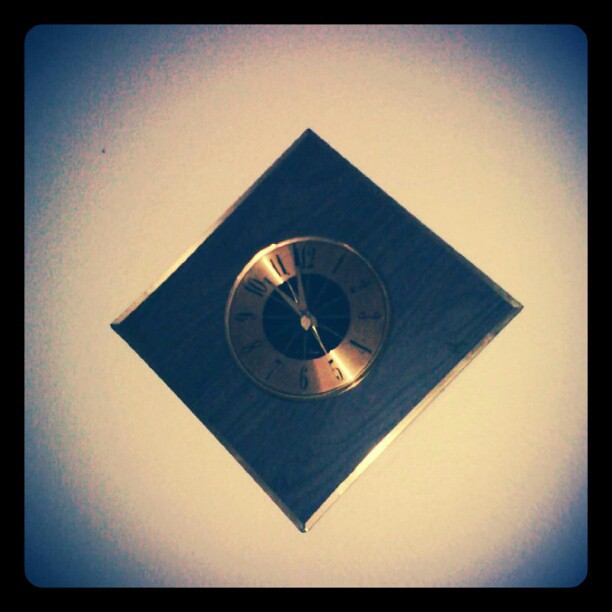The image depicts a low-quality photo of a clock, likely taken with an old phone camera around 10 years ago, characterized by a heavily filtered Instagram-like style. The photo has a black border with curved edges and varying shades of dark purplish-blue splotches at the corners, giving the impression of a camera flash lighting up the wall behind. The clock hangs against a dark wooden background and features a unique design: it is set within a diamond-shaped square frame. The actual clock face is circular with a gold center, potentially adorned with a sun-like design. The clock's numbering from 1 to 12 is in standard black, but due to the photo's fuzzy quality, it is challenging to discern exact details. Upon closer examination, the hands seem to indicate a time around 10:55, though another voice suggests it might be 12:12. The stylized square frame's corners correspond to the 12, 3, 6, and 9 positions on the clock, enhancing its distinctive appearance.